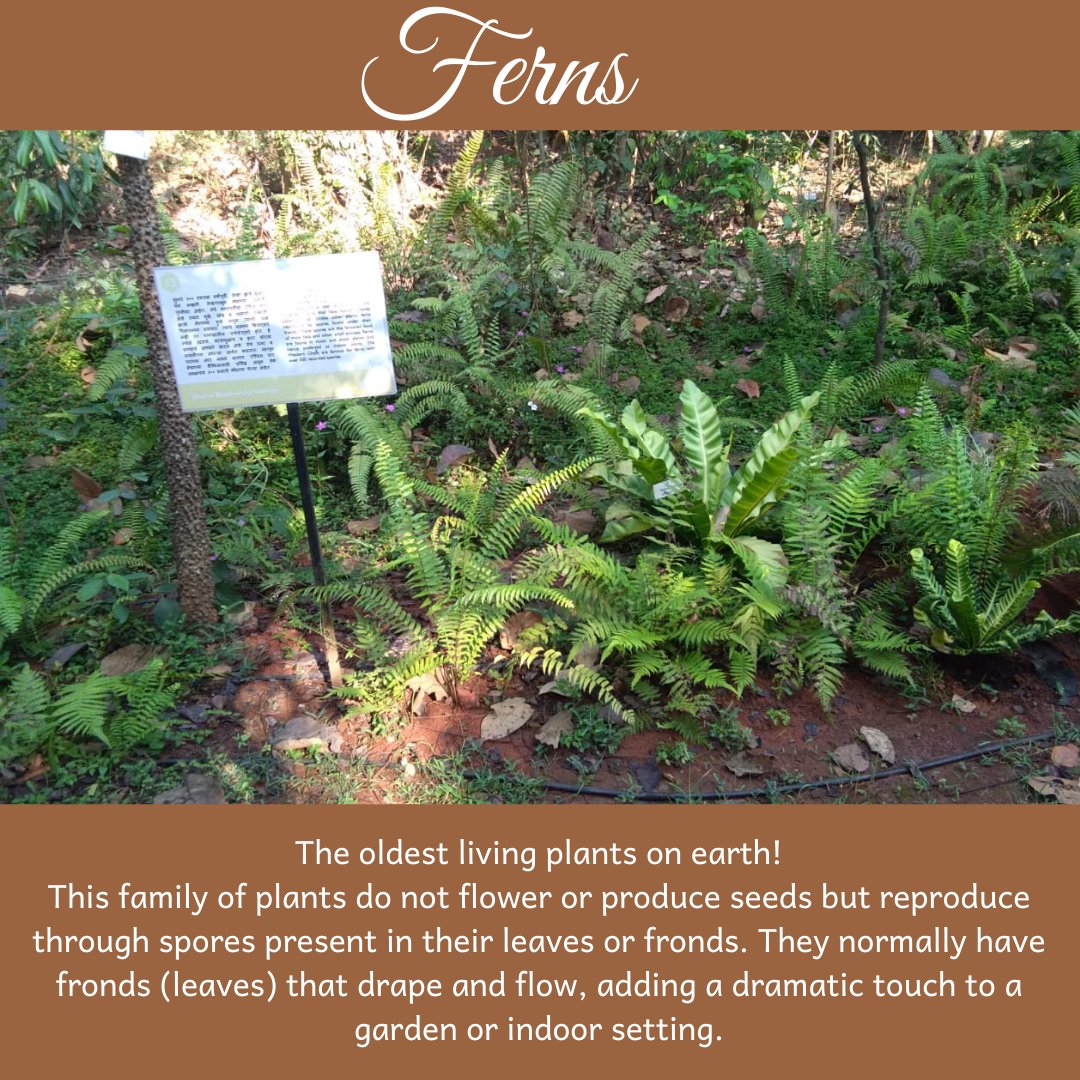In the center of this image, there's a lush collection of green ferns growing from the ground, possibly along a nature trail. The scene is complemented by a variety of plants and grasses, with the soil appearing as a rich brown expanse. On the left side, there's a slim tree trunk beside which stands a signboard. The signboard features a light brown background with text in two sections: the top section reads "ferns" in white cursive font, and the bottom section contains an informative caption in regular white sans-serif font. The caption reads: "The oldest living plants on earth! This family of plants do not flower or produce seeds but reproduce through spores present in their leaves or fronds. They normally have fronds that drape and flow, adding a dramatic touch to a garden or indoor setting." The signboard itself is supported by a black pole and has a small yellow accent at its base.